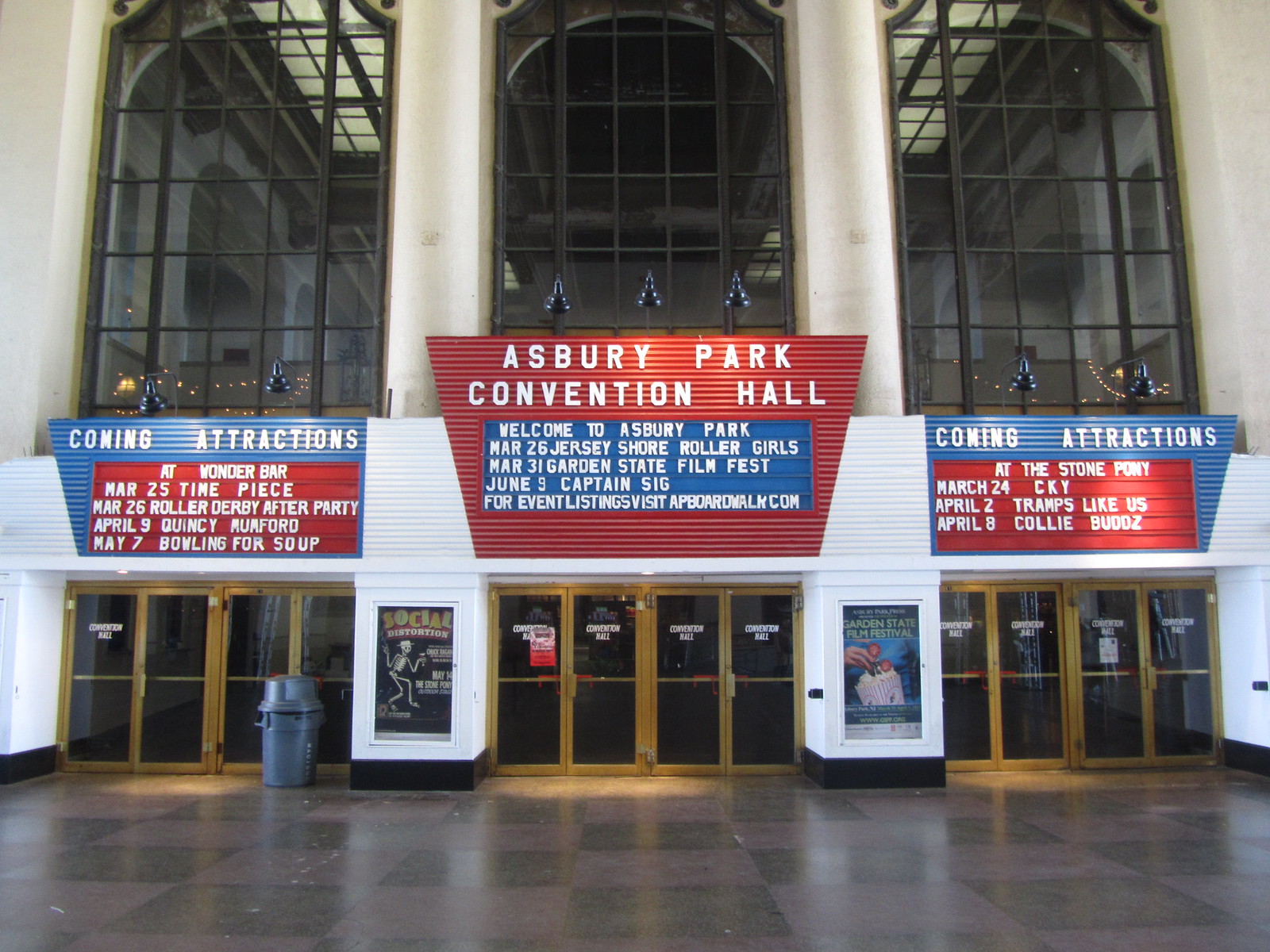The image depicts the front of the Asbury Park Convention Hall, a tall building distinguished by its large, arch-shaped windows divided into rectangular panes by thin bars. The top half of the building features these striking windows, while the lower half showcases white-colored walls with signage. Prominently displayed in the center is a bold, red sign stating “Asbury Park Convention Hall,” above which are gold doors set between white pillars. Below the main sign, a blue banner in white text features welcoming words and a list of events: "Welcome to Asbury Park. March 26th - Jersey Shore Roller Girls, March 31st - Garden State Film Fest, June 5th - Captain Sig Event." Additionally, directional signs above the doors highlight upcoming attractions: on the right, "Coming Attractions at The Stone Pony - March 24th: CKY, April 2nd: Tramps Like Us, April 8th: Kali Buds," and on the left, "Coming Attractions at Wonder Bar - March 25th: Timepiece, March 26th: Roller Derby After Party, April 9th: Quincy Mumford, May 7th: Bowling for Soup." The ground in front of the building is adorned with dark tiles, adding to the overall aesthetic of this event-centric landmark.